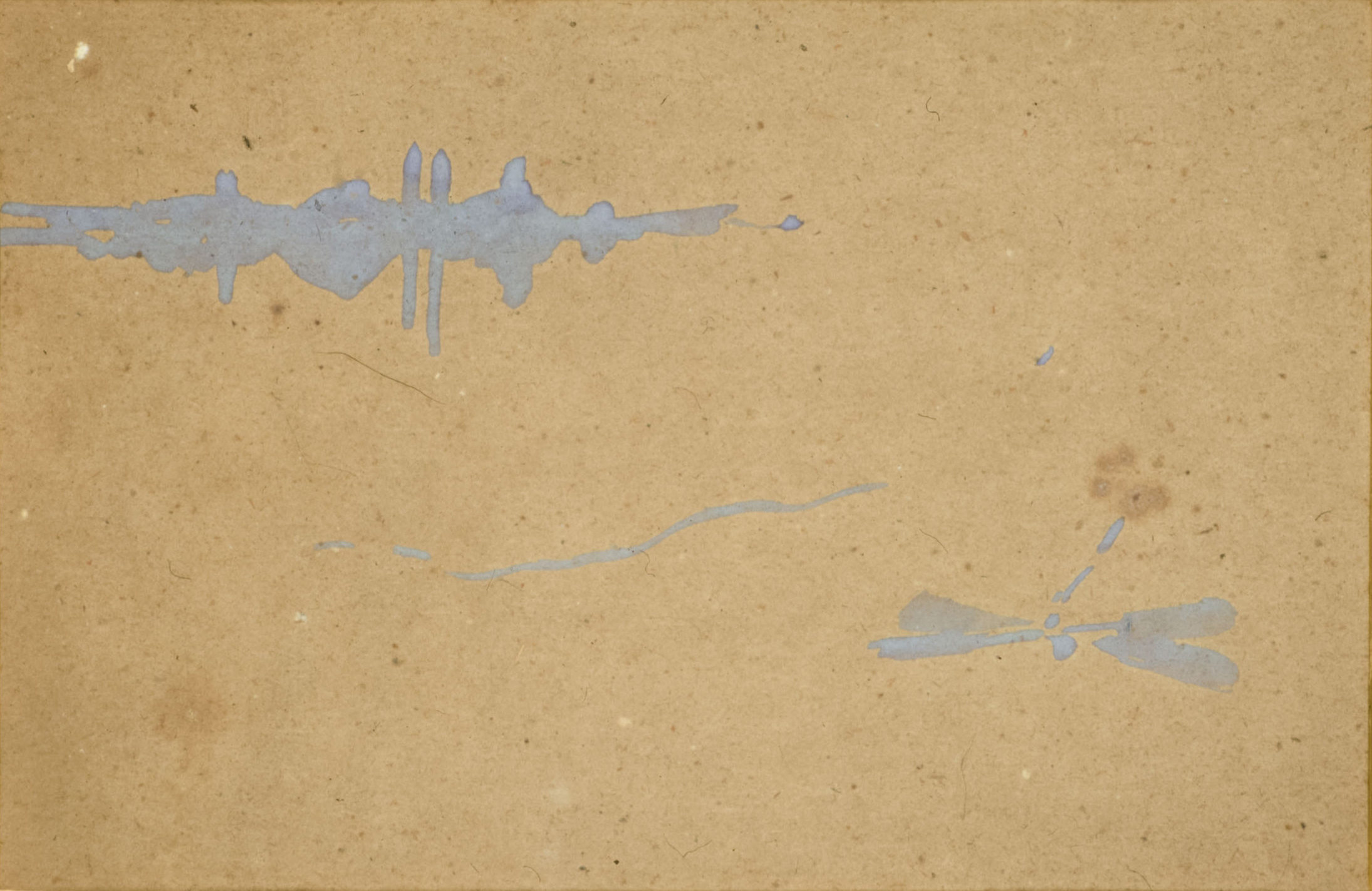This image features a predominantly light brown, rectangular surface that fills the entire frame. The surface, likely a canvas, displays a variety of dark brown spots scattered across it, most of which are small, with a few larger spots near the bottom left corner and the right side. Adding to the textured and abstract nature of the image, there are notable areas of gray. In the top left, a grey patch forms a strange, abstract shape, accompanied by a horizontal and a few vertical streaks of blue, as well as some splotches. A faint grey line runs through the middle of the image. On the bottom right, a gray area intriguingly resembles the shape of an insect with wings, reminiscent of a dragonfly or a butterfly. Additionally, near the top left, just above the gray patch, there is a noticeable white spot. The image lacks context, as there are no visible edges or frames to indicate whether this might be a painting, a floor, or a wall, emphasizing its abstract and textured characteristics.